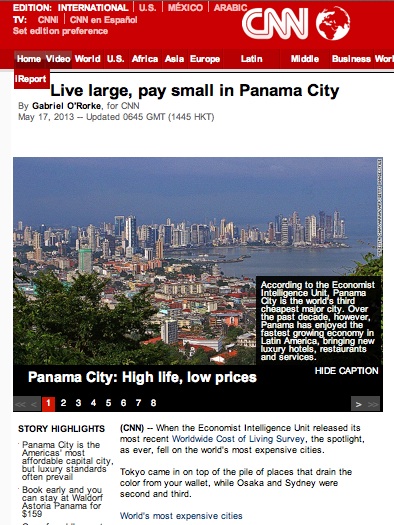A screenshot from an older version of the CNN website reveals a detailed article titled "Live Large, Pay Small in Panama City" by Gabriel O'Rourke, published on May 17, 2013, and updated at 0645 GMT (1445 HKT). The CNN logo is prominently displayed at the top of the page. The website's interface appears dated, featuring a navigation bar with options such as Home, Video, World, U.S., Africa, Asia, Europe, Latin America, and Business World. The edition is set to International, with further preferences encompassing U.S., Mexico, Arabic, and Español versions.

The article discusses the economic transformation of Panama City, which includes an image showcasing the city's bay area lined with numerous skyscrapers. The caption under the image cites the Economist Intelligence Unit, noting that Panama City is the world's third cheapest major city, despite having the fastest-growing economy in Latin America over the past decade, leading to the emergence of new luxury hotels, restaurants, and services. The page also indicates that the article spans seven different pages for those interested in further details.